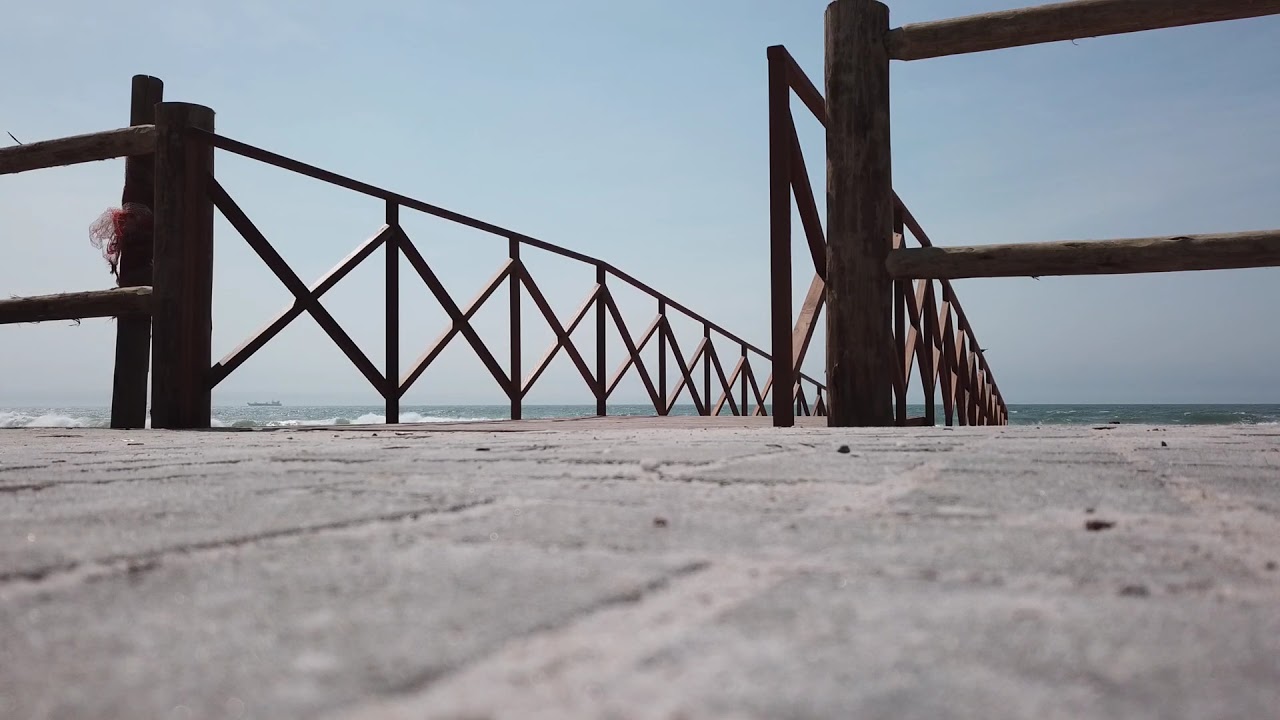This is a photograph taken on a bright, clear day from a ground-level perspective, almost as if the camera is placed directly on a paved, concrete walkway. Centered in the image is a wooden dock with brown horizontal and vertical wooden railings on either side, flanking a brown metal railing that extends outwards, seemingly over the water. The dock appears to dip down at the far end, leading towards the horizon. The ocean, a mix of dark blue and dark green, is visible beyond the railing, with waves gently breaking on the left. The sky above is a clear blue, providing a serene backdrop. The image captures the junction of the walkway, the wooden and metal bridge-like railing, and the open ocean, evoking a tranquil, coastal atmosphere.